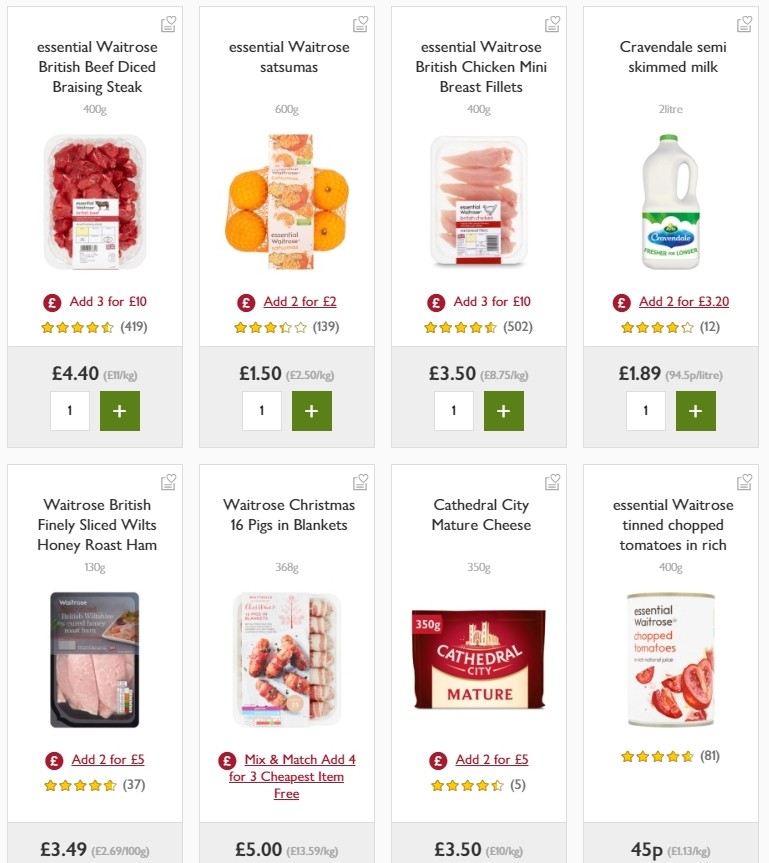This screenshot features a light gray background and displays a layout of grocery items. At the top of the image, there are four vertical rectangles aligned horizontally across the screen. Each rectangle contains detailed information about a specific item.

First, within each rectangle's header, the item name is written in black text at the top center. Below the name, there is a corresponding image of the item. Beneath the image, there are star ratings indicating customer reviews, followed by red text suggesting promotion details like "Add 3 for $4."

At the bottom of each rectangle, in a gray box, the price of the item is clearly displayed. To the left within the gray box, there is a white square outlined in gray containing the number "1." Adjacent to this, on the right side, there is a green square with a white plus sign, which allows users to adjust the quantity of the item.

In the section below the first set of items, the gray boxes containing the prices are mostly visible, though partially cut off. Nonetheless, it's clear that the layout continues to follow the same structure.

The displayed items include common grocery store products such as oranges, chicken breast fillets, milk, ice cream, and honey-roasted ham, each with their respective images, prices, and quantity adjustment options.